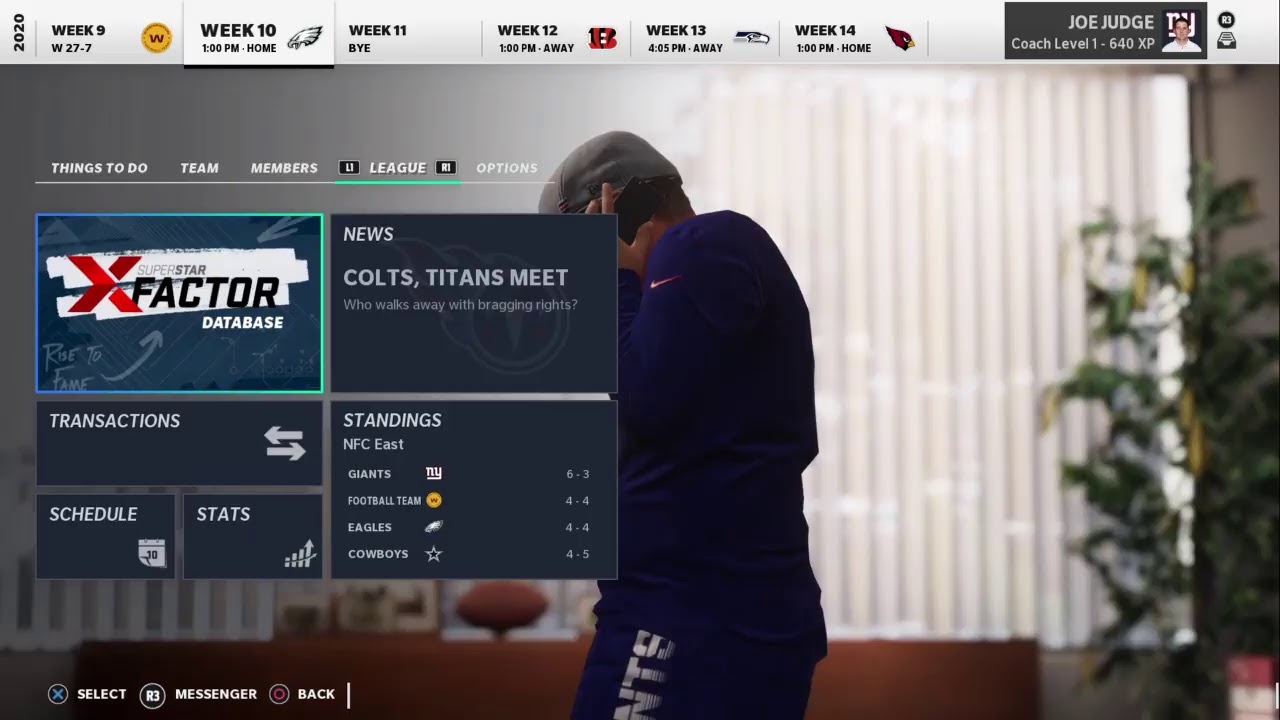This image showcases a detailed screenshot of a sports website, likely dedicated to a football league. The central part of the page prominently features a person dressed in a matching track suit, complete with a gray cap, and appears to be on the phone. His face is obscured by an overlay of schedules and stats, adding a dynamic element to the scene.

The top section of the website includes navigational tabs labeled "Things to Do," "Team," "Members," "League," and "Options," with additional headings for "News," "Cults," "Titans," and a debate about which team will walk away with bragging rights. Further below, the page offers options for accessing "Transactions," "Schedule Stats," and a "Standings" box listing teams: Giants, Football Team, Eagles, and Cowboys. Another section prompts the user to "Select Messenger Back."

On the left side, there is a photograph of Joe Judge, a white coach prominently displayed under a title reading "Coach Level One" dated for the year 2020. The schedule for the season is divided into weeks 9 through 14, each represented by distinct images and elements: a ‘W’ for week 9, a feather for week 10, with week 11 marked as a bye-week. Week 12 features a home and away schedule, week 13 another unidentified image, and week 14 repeats the feathery motif.

The scene suggests an office or home setting, showing a red couch, a plant, and a football on display, providing a personal touch to the environment. The entire composition paints a comprehensive picture of the website’s user interface, offering insights into football season planning and fan engagement elements.